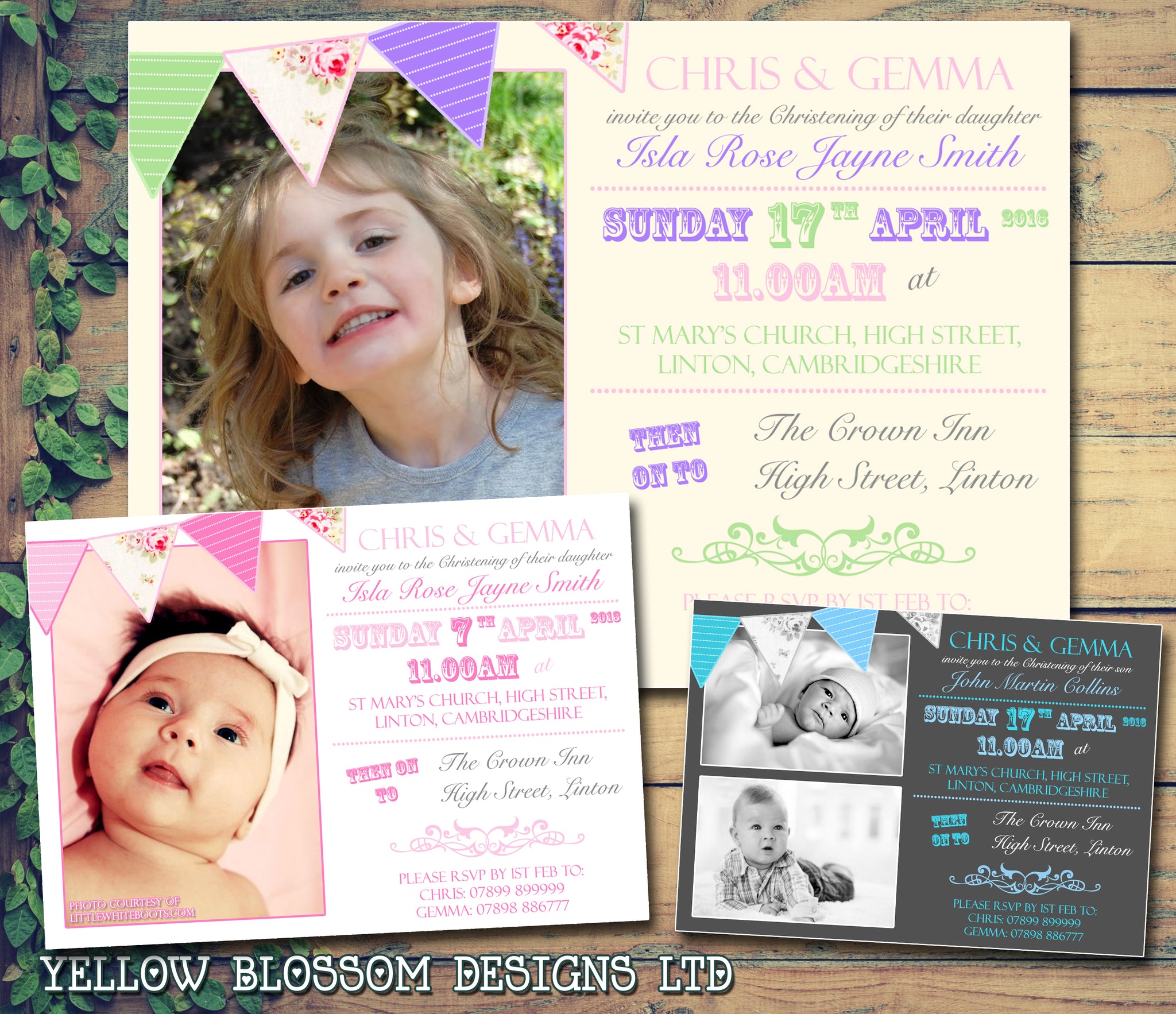The image features three distinct announcements or invitations set against a brown wooden table with planks running horizontally and adorned with small ivy leaves cascading down the left side. The announcements are christening invitations from Yellow Blossom Designs Limited, elegantly labeled in white cursive text at the bottom left of the image.

At the top, a large cream-colored card with pink, purple, and green text invites guests to the christening of Chris and Gemma's daughter, Isla Rose Jane Smith. This event is scheduled for Sunday, April 17, 2016, at 11 a.m. at St. Mary's Church on High Street in Linton, Cambridgeshire, followed by a reception at The Crown Inn, also on High Street in Linton. The card includes an RSVP request by February 1st.

To the bottom left, there's a smaller white card with pink accents for a baby girl's christening, while a gray and blue card on the bottom right announces the christening of Chris and Gemma's son, John Martin Collins, on the same date and time as Isla's, with the same venue details. Each card prominently features respective photographs of the children, integrating a personal touch. The design and cohesive presentation of the invitations emphasize the creative branding of Yellow Blossom Designs Limited.